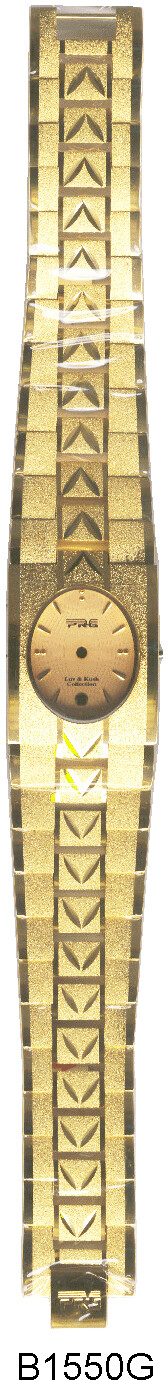Here is a refined and detailed caption for the illustration based on the provided description:

---

**Illustrated Gold Decorative Watch on White Background**

This color illustration depicts an elegantly designed, decorative watch with a predominantly gold theme. Set against a pristine white backdrop, the watch appears prominently featured, suggesting a tall and narrow composition, as it is closely positioned near surrounding text.

The watch itself boasts an oval face in a rich, dark gold hue. Instead of traditional numerals, small markers denote the hours. Notably, the illustration does not display the watch hands, which might be an artistic choice or an oversight. Two tiny logos, one positioned at the top and the other at the bottom of the watch face, are present but too minuscule to decipher.

Attached to the watch face is an exquisite gold bracelet, adorned with intricate triangular patterns that point upwards and downwards, adding an extra touch of sophistication. This bracelet features an outer band composed of square or rectangular links, lending it a structural charm. The band’s width dynamically adjusts, being broader near the face and tapering off towards the ends where it securely fastens with a clasp.

At the bottom of the illustration, the code "B15550G" is inscribed in black, likely serving as a model or identification number for the watch.

---